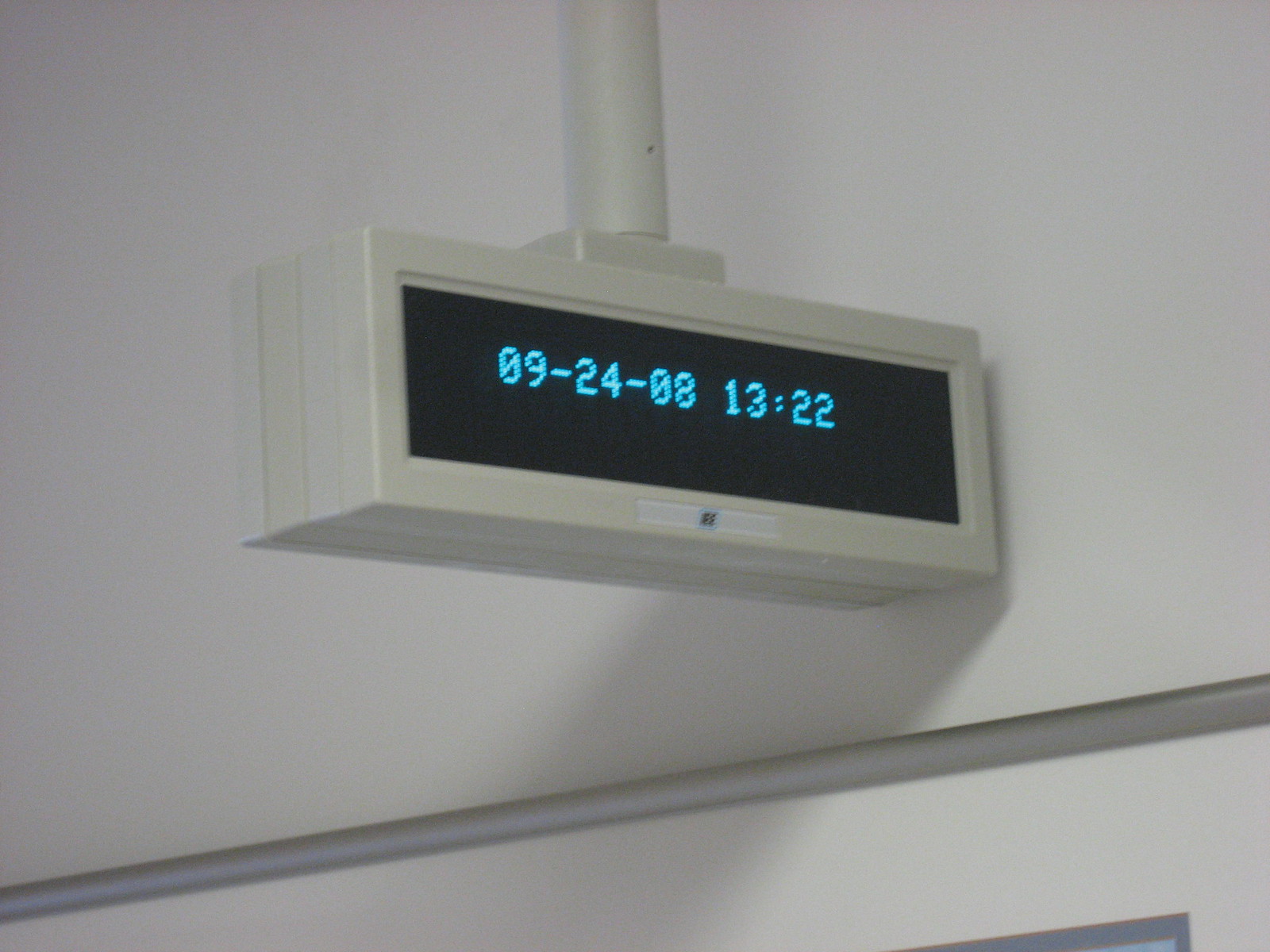The image depicts a digital sign suspended horizontally from a white wall. This rectangular sign is encased in white plastic and features a black screen displaying blue numbers indicating the date, "09-24-08," and time, "13:22" (1:22 p.m.). Beneath the sign, there appears to be a silver frame rather than a door. In the foreground, a gray bar runs across the photo from the bottom left to the bottom right, with a partial piece of another gray bar underneath. The background of the photo is white, adorned with white walls and a white door frame. Additionally, a shadow cast by the light source falls on the wall below the digital sign, contributing to the overall composition. In the bottom right corner of the image, there is a small section of a gray map or photo visible within the frame.